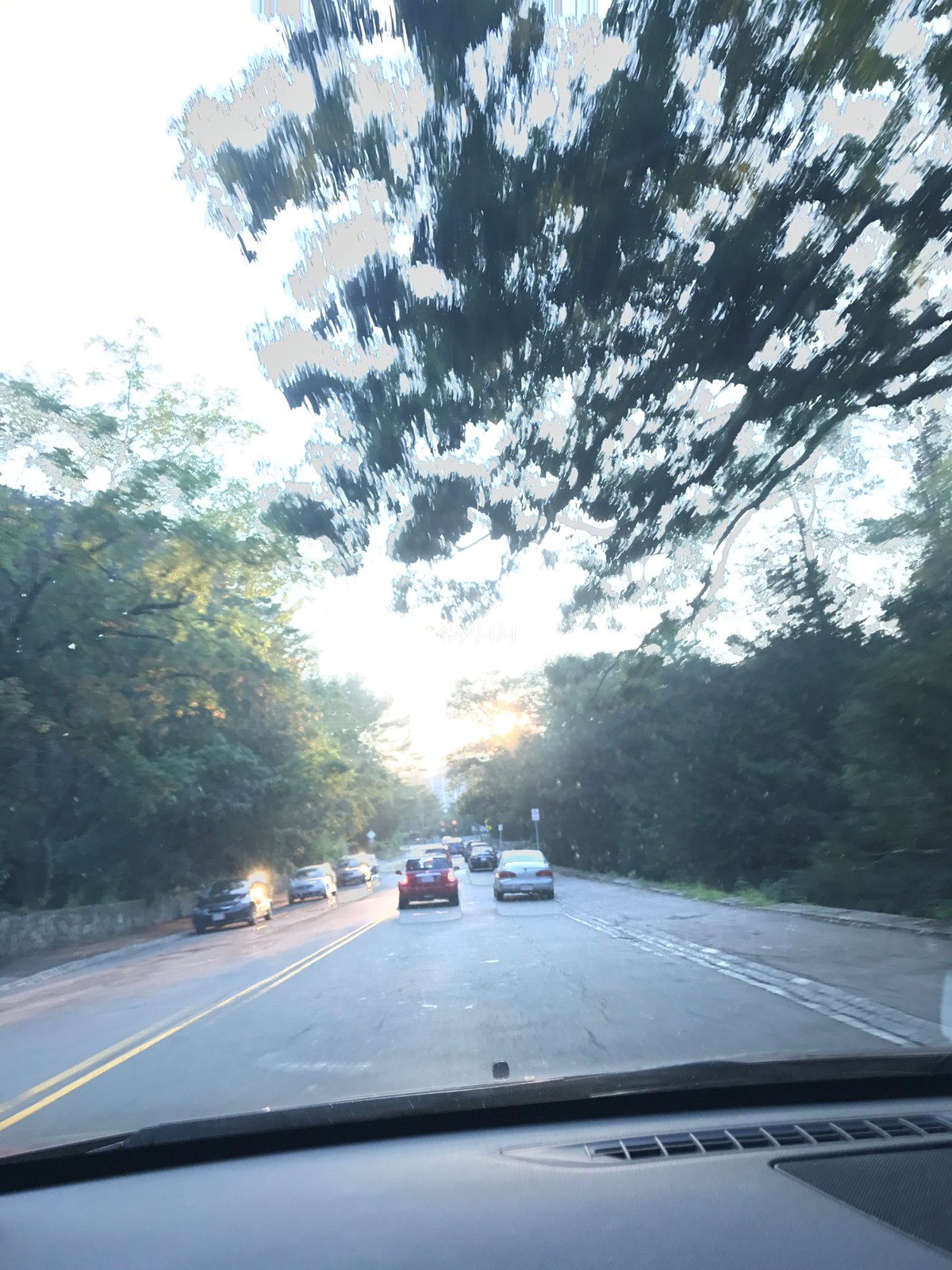The photo, captured from inside a car through the front windshield, provides a vivid glimpse of a road scene. Visible inside the car is a section of the air vent, framing the view ahead. The car is traveling down a two-lane road, each lane separated by a double yellow line. On the right-hand side, a sidewalk runs parallel to the roadway. In front of the car are two vehicles: a small red car followed by a silver Toyota Corolla, the latter appearing to straddle the middle of both lanes. Both sides of the street are lined with trees, adding a leafy canopy to the scene. On the left-hand side, beyond the sidewalk, a stone wall runs along the street, with a row of four parked cars adding to the urban tableau.